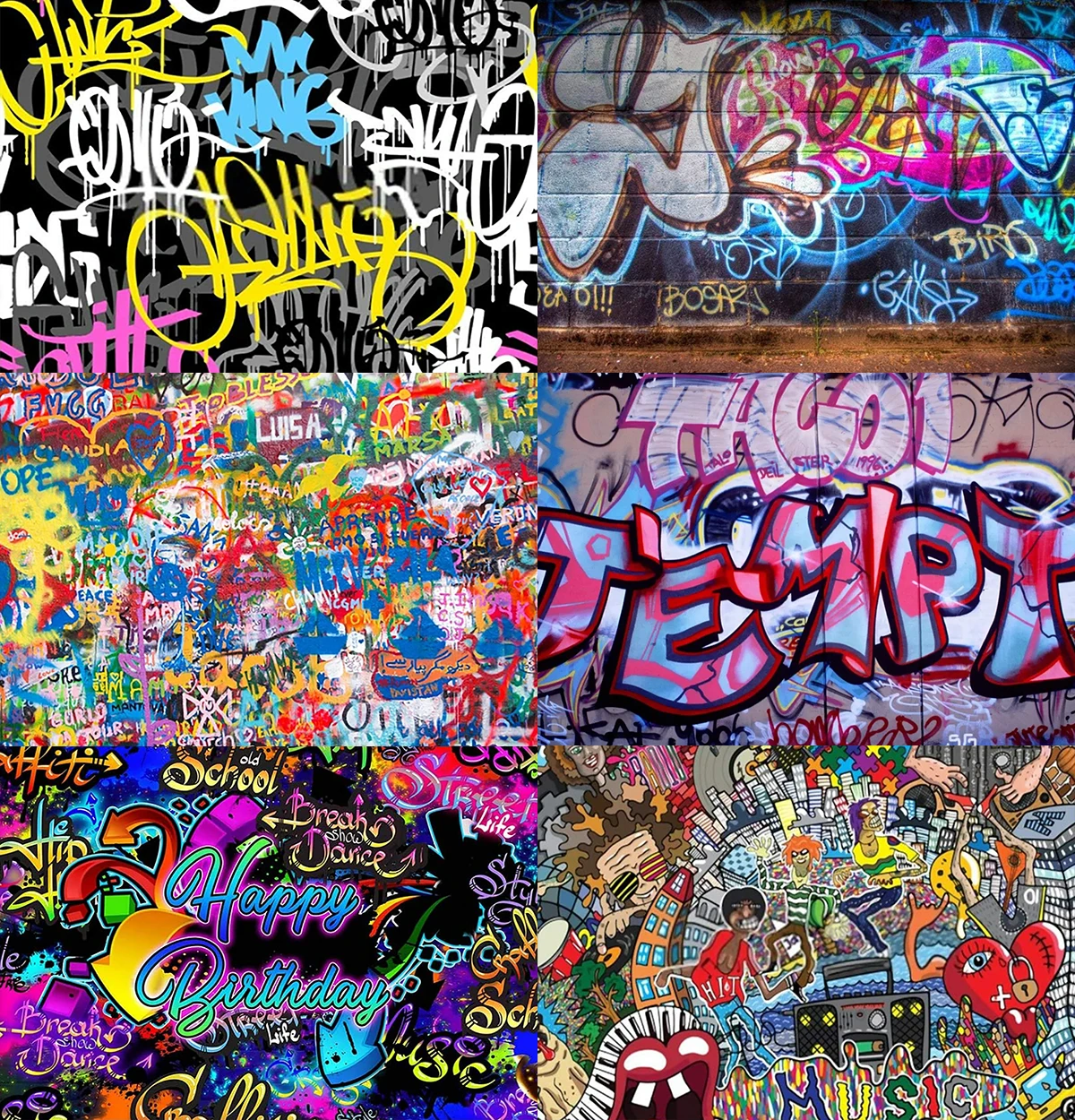This image is a vibrant collage of six graffiti or street art panels, arranged in two columns and three rows. The top left panel showcases a black wall adorned with a chaotic blend of yellow, white, blue, and pink graffiti letters or words. The top right panel continues the theme with another black wall featuring a large letter 'J,' intermingled with blue, pink, white, and green colors. The middle left panel is a dense scramble of various colorful words and names, obscuring the wall beneath them. Opposite to this, the middle right panel prominently displays the word 'TEMPT' in striking pink font. The bottom left panel celebrates with a 'Happy Birthday' message in bold blue letters accompanied by green accents against a black backdrop. Finally, the bottom right panel diverges slightly, depicting a vibrant cityscape complete with buildings, characters, and a prominent word 'MUSIC,' rendered in an array of lively colors. Overall, the collage is a dynamic and colorful testament to the expressive nature of street art.